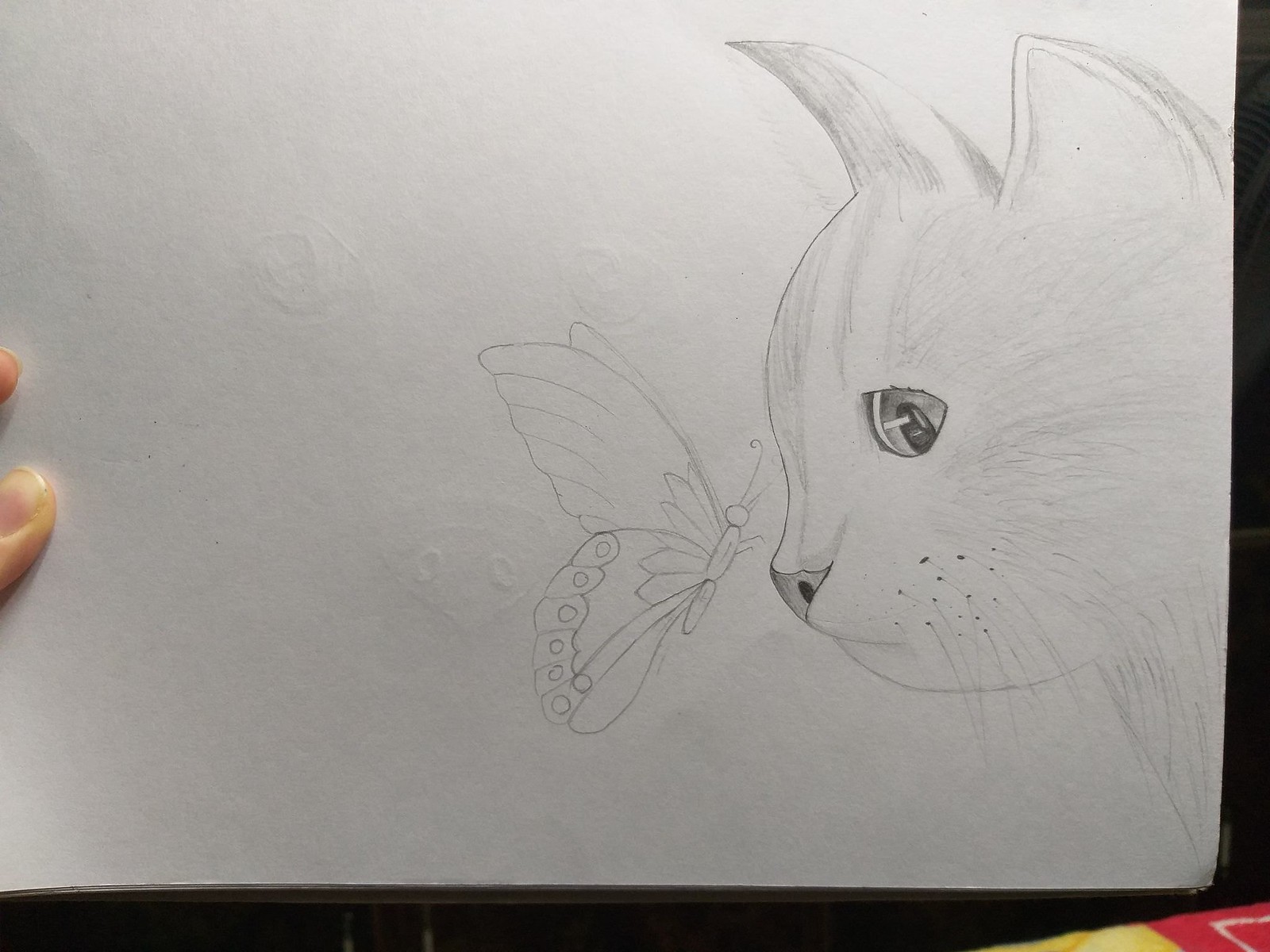The image captures a stunning pencil sketch of a kitty, meticulously detailed yet minimalist in execution. The cat’s eye, a focal point, is rendered with intricate care, showcasing glistening reflections that lend it a glassy, lifelike quality. The fur, whiskers, and ear curvature are depicted with a few precise lines, creating a strikingly realistic and captivating portrait. Perched delicately near the cat’s nose is a beautifully sketched butterfly, composed of minimal lines yet exuding elegance and simplicity. The kitten gazes intently at the butterfly, creating a moment of quiet interaction. To the left side of the sketch, the artist's two fingers are partially visible, hinting at the process behind this exquisite artwork. The background is primarily gray, with a distinct black area framing the edges of the paper, enhancing the composition’s overall minimalistic beauty.